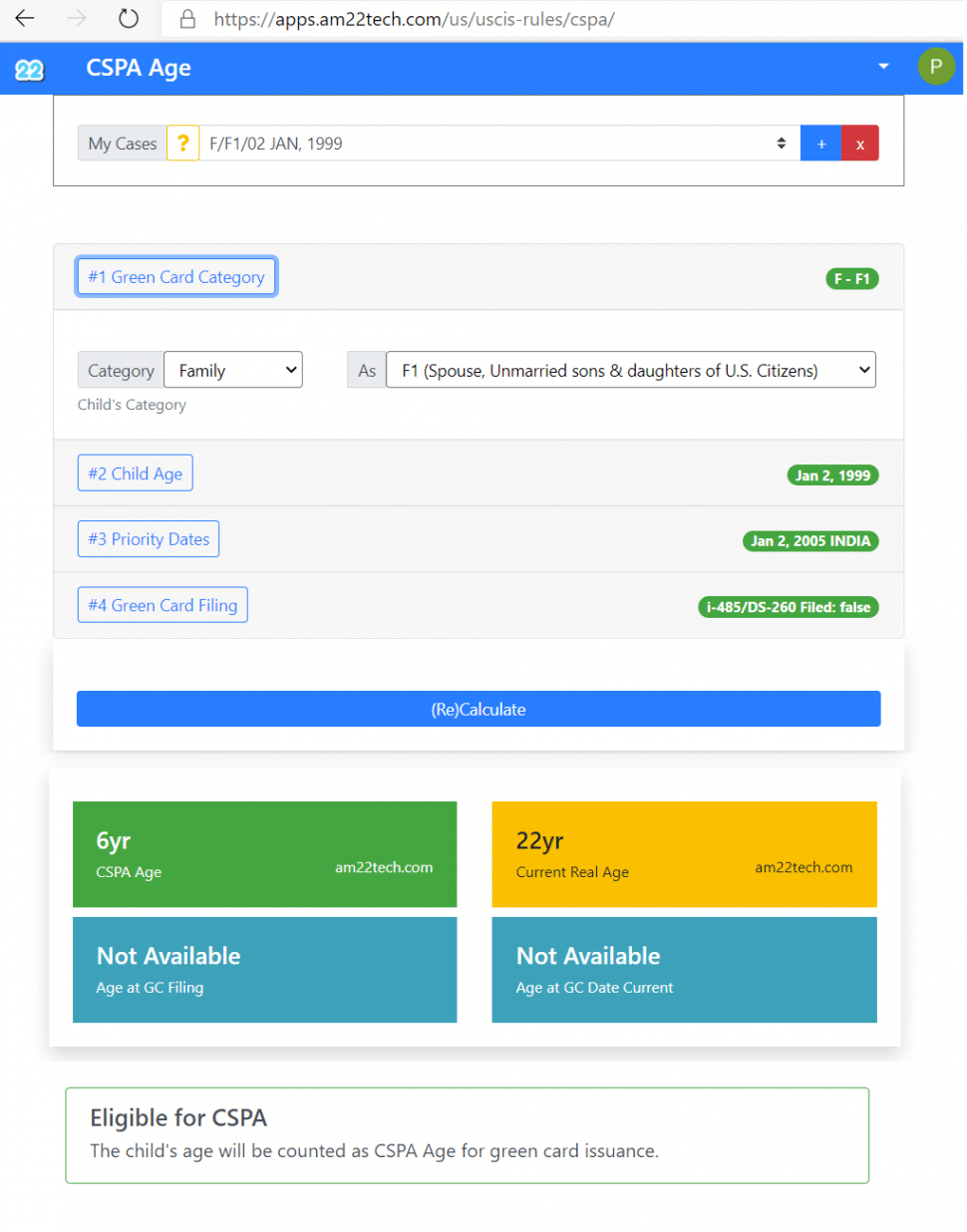Here is a cleaned-up and detailed caption for the image described:

---

The image displays a complex graphical chart, starting with navigation symbols on the top left corner including a left arrow, a right arrow, and a rotating icon. Beneath these icons, a URL reads "https://apps.tech.com.us.cis-rules.cspa." 

The chart features a prominent blue border labeled "CSPA Age," with a green circle at the bottom of this segment detailing a case identifier, "?f.f102.Jan.2009". The background beneath these elements alternates in blue, red, and white colors.

The next segment is framed by a border stating "Number One Green Card Category," and contains further details such as "F-something, Category: Family, Child's Category". A list of categories follows, including "F1, Spouse, Unmarried Sons and Daughters of U.S. Citizens."

Three key points are highlighted:
1. "Child’s Age: Jan. 2, 2009,"
2. "Priority Date: Jan. 2, 2005, India,"
3. "Green Card Filing Status."

Moving further down, the chart showcases several colored squares:
- A blue rectangle indicating "Recalculate,"
- A green square with "Six-Year CSPA Age,"
- A yellow square with "22-Year Current Real Age."

Finally, another blue rectangle notes "Not Available Age" for both "GC Filing Date" and "Current". The bottom-most detail confirms whether an individual is "Eligible for CSPA Age" regarding green card issuance, all set against a plain white background.